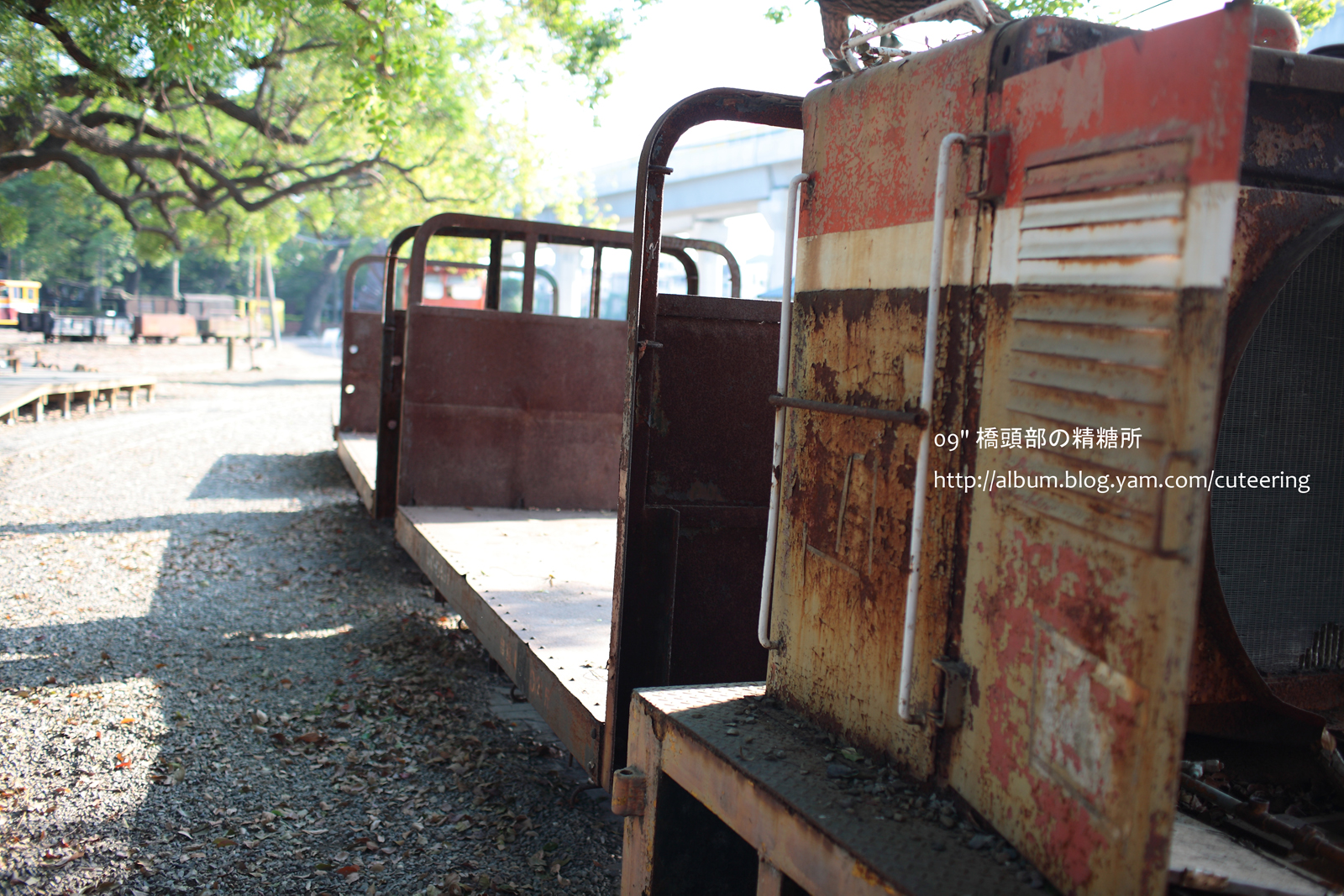The outdoor image showcases a vibrant, sunny sky accented with white clouds and dense green foliage from a row of trees in the background. In the mid-ground, a partial view of tree branches with lush green leaves is visible. The setting features a gravelly ground that supports various metal platforms and contraptions. Prominently, a low wooden deck stretches across the scene, bordered by what seems to be abandoned train cars or storage containers, spaced apart without wheels, and exhibiting a blend of white and rusted metal surfaces. These containers have red and white stripes and rusted handles, indicating significant wear and age. In the extreme foreground stands an aged metal structure with a combination of brownish rust and maroon hues, possessing railings and a metal door or ventilation system. The right side of the frame also includes a credit mark reading "09” with Japanese symbols, a web address, and the year 2009, adding an aura of mystery to the intriguing, abandoned landscape.